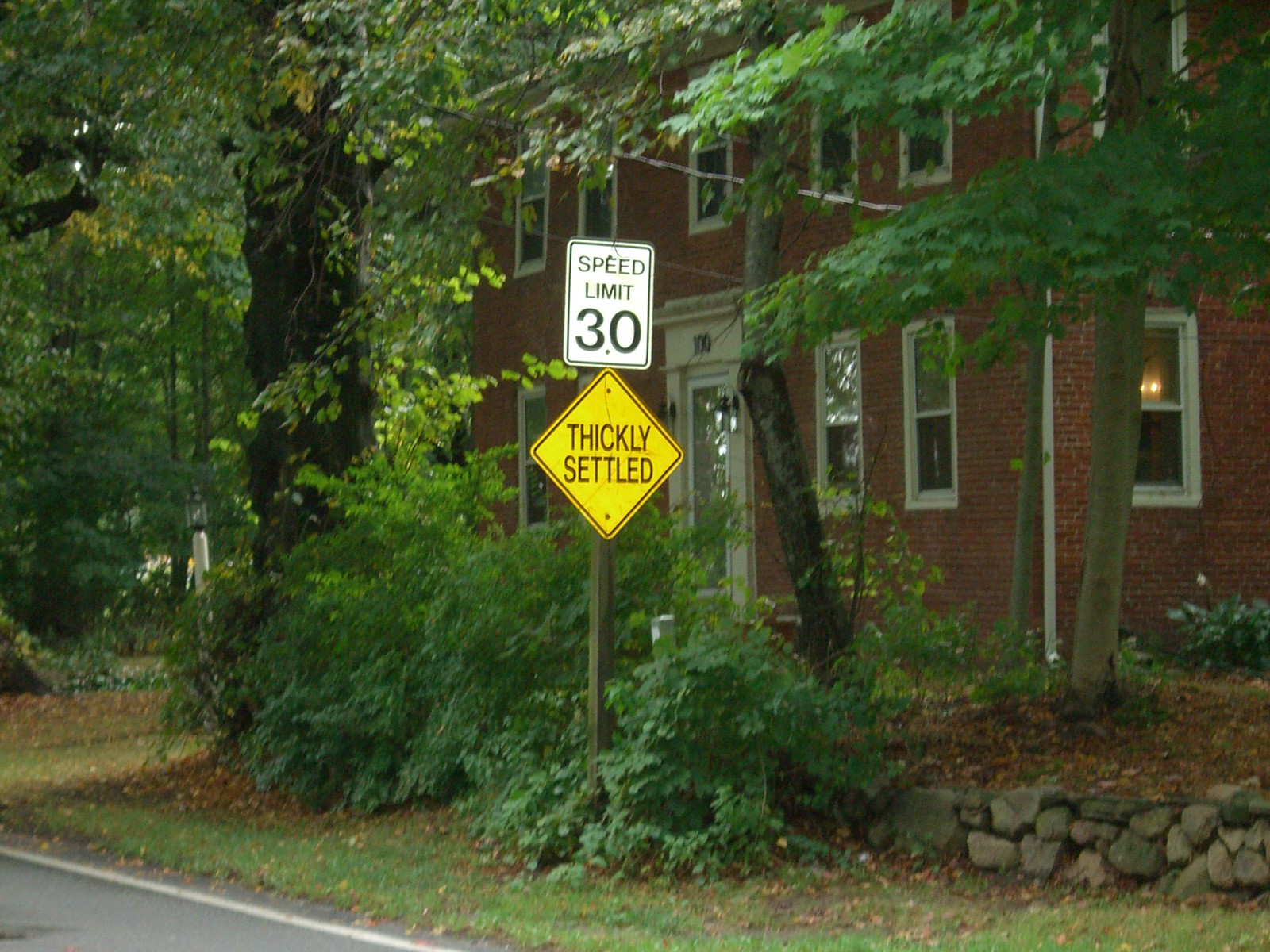This photograph captures a scene along the edge of a road, where nature and man-made structures intertwine. In the center of the image, there is a prominent speed limit sign, a white rectangular sign with black lettering that indicates a speed limit of 30. Directly below the speed limit sign, a yellow diamond-shaped sign with black writing warns "Thickly Settled." Both signs are mounted on a post, either metal or wooden, firmly planted in the ground.

Surrounding the signpost, dense bushes and overgrown foliage create a lush foreground. Taller trees rise behind these bushes, their branches reaching towards the sky, partially obscuring a brick building in the background. The building is constructed from reddish bricks and features large white-framed windows. Above the entrance, the number "100" is prominently displayed.

In the lower right-hand corner of the photograph, a short, low stone wall is visible, with grass and dirt in front of it. A solitary tree stands behind the wall, its trunk and branches extending upwards. The lower left-hand corner of the image reveals a small glimpse of the road, providing context to the otherwise secluded scene. The overall composition blends architectural elements with the natural environment, creating a peaceful yet slightly overgrown roadside vignette.